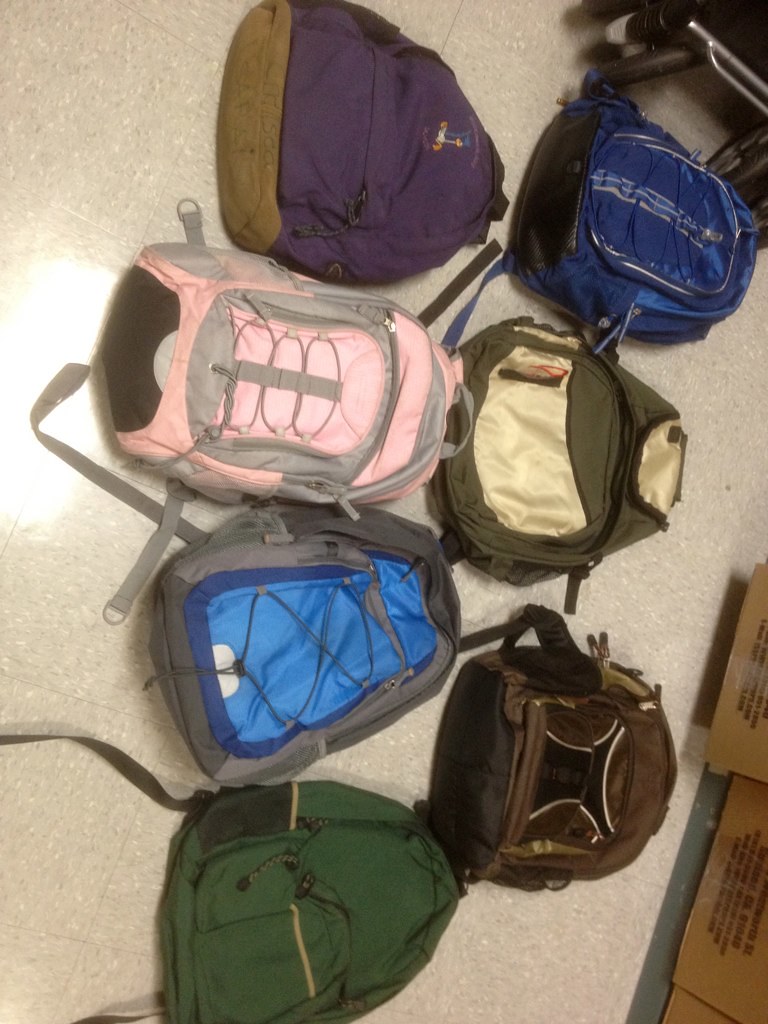This digital photograph, likely taken indoors, features seven colorful backpacks arranged vertically in two columns on a multicolored tiled floor resembling what you might find in an American classroom. The tiles are predominantly tannish-brown with lighter and darker speckles. In the upper right corner, there's a black device with black wheels, and the bottom right shows partially cropped tan boxes with black writing. The backpacks, all lying flat, are:

1. A purple backpack with a brown bottom (top left).
2. A grayish-silver backpack (middle left).
3. A pink backpack with a black bottom (middle left).
4. A blue backpack with a gray outline (middle right).
5. An olive-green backpack with a white patch on the pouch and top (middle right).
6. A dark brown backpack with a black bottom and an X-shaped design (bottom right).
7. A green backpack with a brown stripe (bottom left).